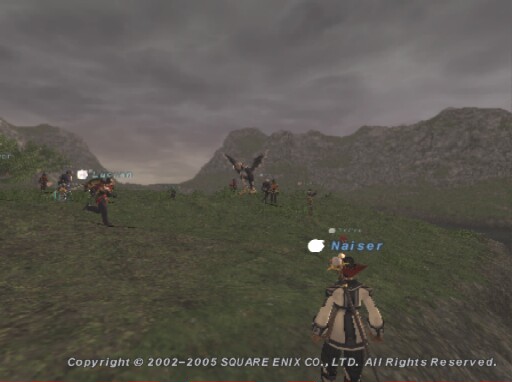This is a screenshot from the original multiplayer game in the Final Fantasy series, reminiscent of early 2000s graphics. The scene features a grey, cloudy sky hovering over a basic, green terrain. At the bottom of the image, a white font displays the copyright notice: "© 2002-2005 Square Enix Co., Ltd. All Rights Reserved." Right above this text, a small avatar representing the player is visible, adorned in a white and blue wizard-like outfit. In the distance, a majestic griffin is seen flying while other players are scattered and running around, adding life and activity to the scene.